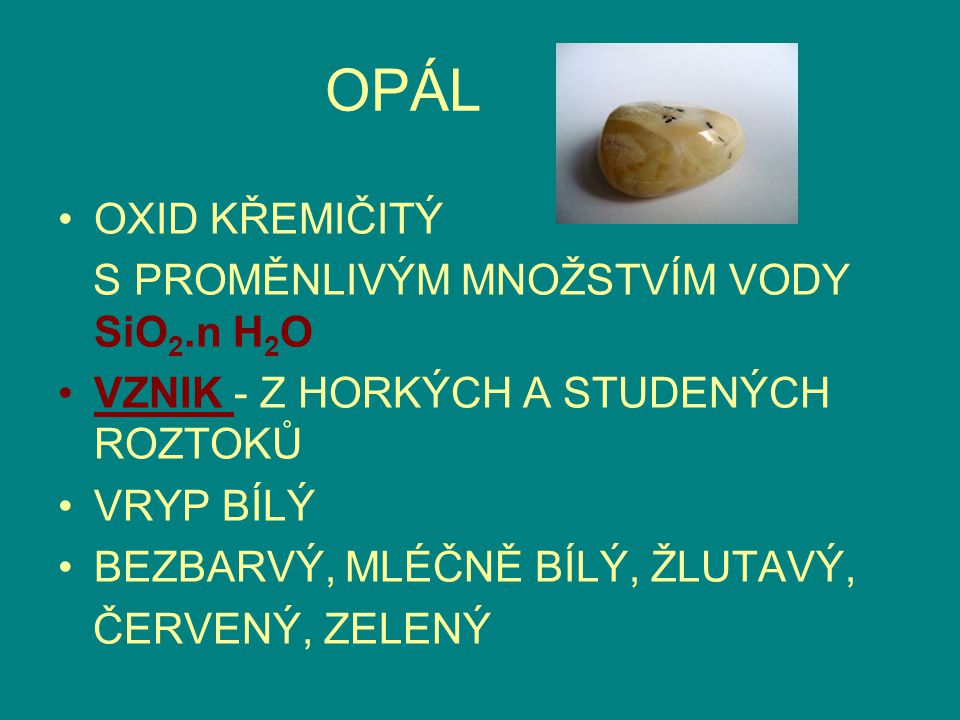The slide features a turquoise or teal background and is predominantly in a language that is not identifiable. At the top, in light yellow font, is the heading "Opal." To the top right of this heading, there is an image of an oval-shaped, shiny light brown rock with varying shades of light brown, set against a white background. Beneath this, there is a bulleted list consisting of four points. All the bullet points are in yellow font except for the second one, which is in red font, underlined, and reads "VZNIK." The first bullet point contains a formula: "SiO2.nH2O," indicating the chemical composition of opal.